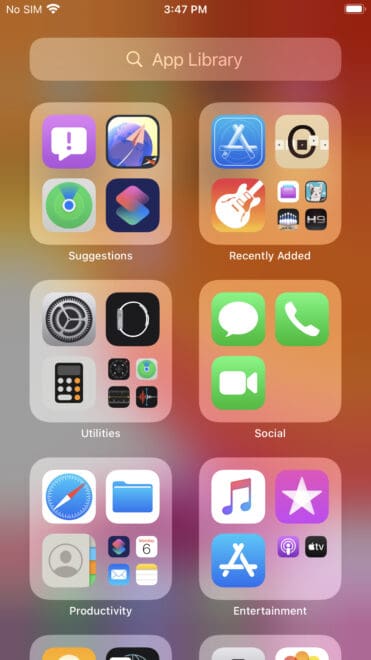This image is a detailed screenshot of a smartphone's App Library. Along the top of the screen, the status bar displays "No SIM" and a Wi-Fi signal icon on the left, "3:47 PM" centered, and a battery indicator on the right. The wallpaper is a blurred reddish tone, making it indistinct.

At the very top, there's a search bar labeled "App Library." Below this, the first row contains two app groups. The leftmost group is titled "Suggestions" and includes apps like Find My iPhone and Shortcuts. To its right is the "Utilities" category, showcasing apps such as Apple Watch, Calculator, Find My, Voice Memos, and Settings.

In the next row, three more app groups are visible. "Social" contains Text, Phone, and Videos apps. "Productivity" includes Email, Internet, Contacts, Files, and Notes apps. "Entertainment" houses the App Store, Apple Music, Podcasts, and Apple TV apps. There are two additional groups at the bottom of the screenshot, but only the very tops are visible, leaving their contents unspecified.